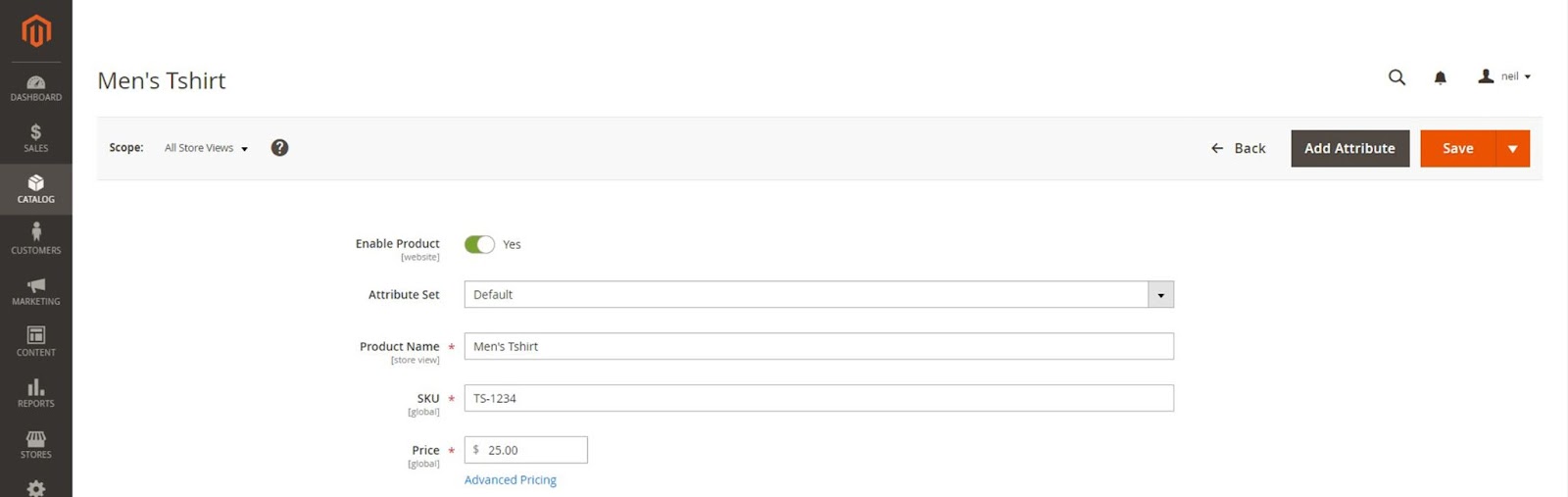The image depicts a detailed interface of a shopping website, likely intended for managing product listings. On the left side of the screen, there's a vertical, dark gray sidebar resembling a minimalist house shape with a "U" inside it. The sidebar contains menu items such as Dashboard, Sales, Catalog (highlighted in a lighter gray), Customers, Marketing, Content, Reports, and Stores.

In the main section, there is a product listing for a Men's T-shirt displayed on a white background. The interface includes options and buttons such as "Scope: All Stores Viewed" and a black circle with a white question mark for help or additional information. There's also a "Back" button labeled plainly as "Back."

Additional interactive elements include "Add Attribute" and a "Save" function within a dropdown highlighted in orange. The "Enable Product" toggle is styled like a pill, with the green part indicating that it is set to "Yes." Below that, configurable fields show the attribute set to "Default," the product name as "Men's T-shirt," the SKU as "TS1234," and the price listed as $25.

The overall layout suggests a distributor’s tool designed for managing the sale of shirts, offering an organized and user-friendly interface for updating product attributes and inventory details.